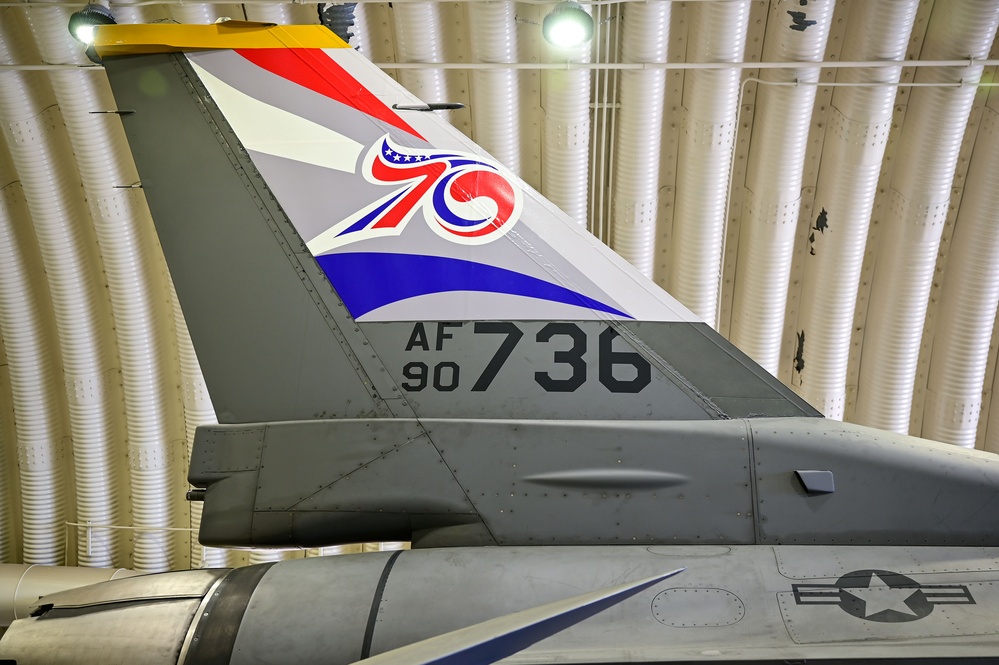The photograph is a detailed, full-color image taken indoors using artificial light. The image is horizontally rectangular without a specific border or background. The ceiling features vertically arranged corrugated white tubes with some wires running horizontally. Across the top, a couple of ceiling lights are visible and illuminated. The photo primarily captures the tail fin of a gray Air Force jet, adorned with the lettering "AF 9736" in black. On the lower section of the tail, closer to the body of the plane, you can see a circular Air Force insignia—a black circle with a white star and two bars like the American flag. The tail fin itself displays a patriotic design: a painted area with red and white stripes and a vibrant red, white, and blue "70," with the '7' in red, the '0' in a mix of blue and red with white stars. Below the tail fin, the jet's powerful booster engine is clearly visible. The aircraft is positioned within what appears to be a hangar, contributing to the industrial and functional atmosphere of the scene.